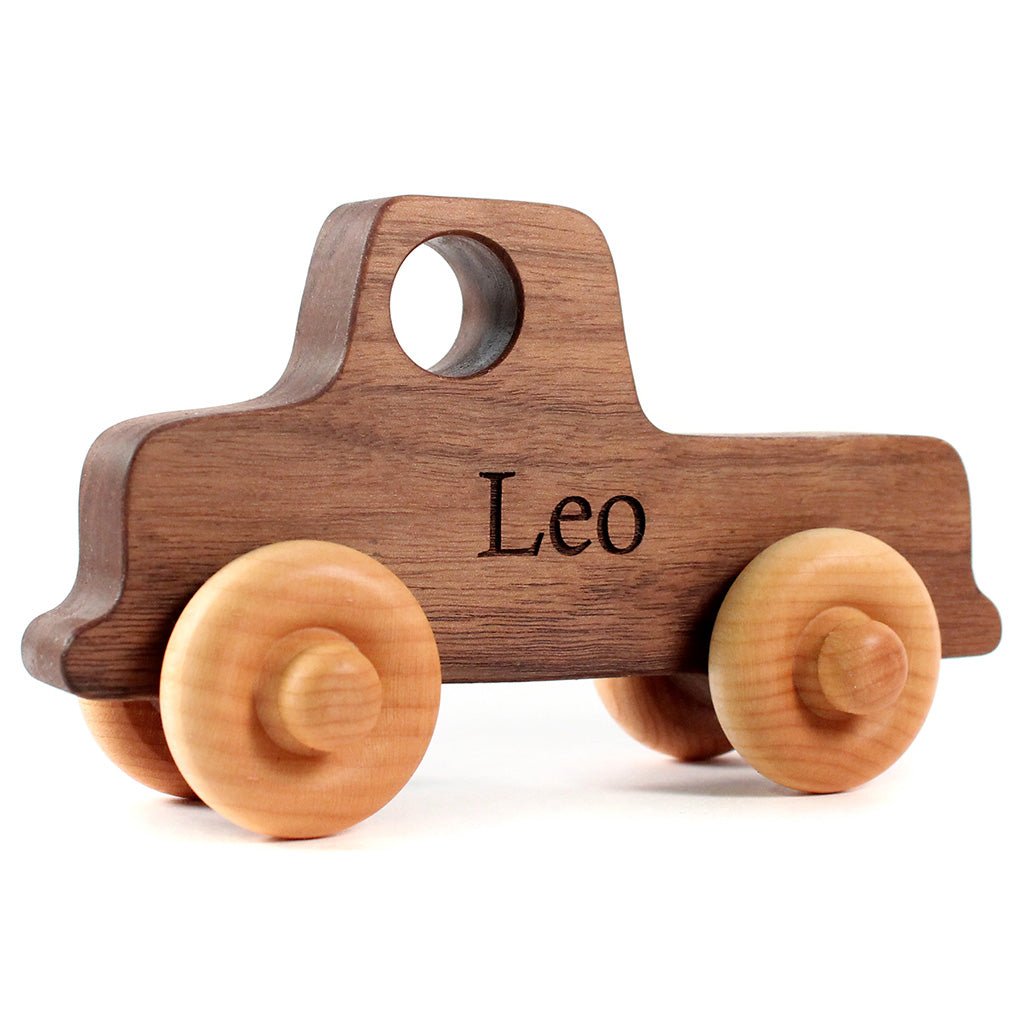The image features a simple, handmade wooden toy truck set against a plain white background. The truck, rendered in a dark-stained wood, has a distinctly crafted appearance, almost hand-carved, with smooth lines and minimalistic details. A single circle hole is drilled into the body to represent the window. The truck's body is stained a medium to dark walnut brown, while the wheels stand out in a lighter, blonde wood, possibly finished with an eggshell or satin sheen, creating a striking contrast. The name "Leo" is engraved into the side of the truck in basic, Times New Roman-like letters, indicating it was made for or given to a boy named Leo. The overall design of the toy is flat and simplistic, embodying the essence of a child's plaything with an understated charm.